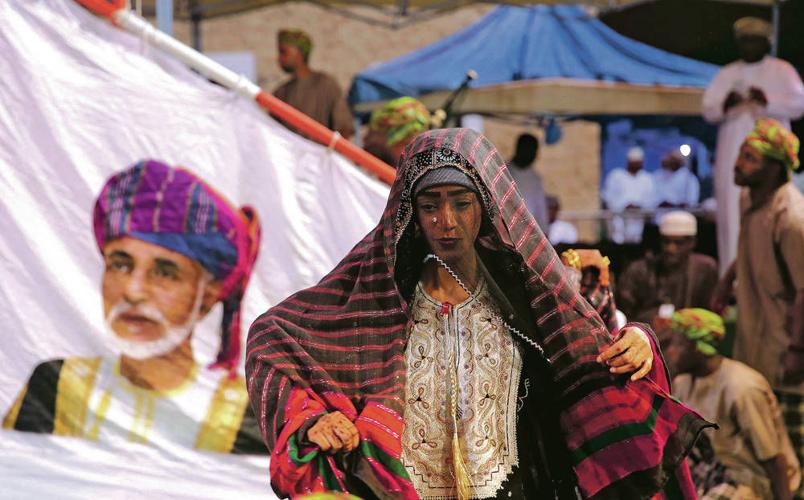In this poignant photograph, a woman with a dark complexion is depicted walking solemnly, seemingly in the midst of a significant ceremony, possibly set in the Middle East. Adorning her head is a large, blanket-like scarf in reddish and black stripes, which partially obscures her tear-streaked face. Her patterned outfit underneath adds texture and depth to her appearance. The backdrop features a striking flag bearing the image of a man with a white beard, dressed in a gold and black ensemble and wearing a turban. Accompanying her in the background are several men, also in traditional attire, including turbans and flowing gowns, adding to the cultural richness of the scene. The woman appears to be walking towards the camera, capturing a candid moment steeped in emotion and cultural significance.